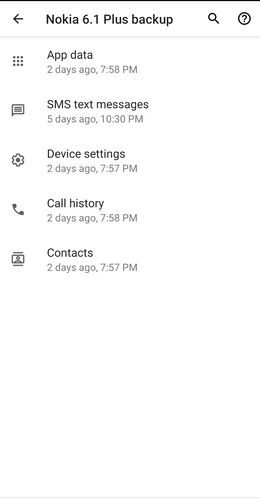At the top of the image, there is a black divider line. Below it, towards the left in dark gray, there is a left-pointing arrow signifying navigability to the previous menu. Centered in bold dark gray text, it reads "Nokia 6.1 Plus Backup." On the right side, there is a magnifying glass icon angled from the lower right to the upper left. Adjacent to it, there is a dark gray circular icon with a question mark in the center, indicating help.

Beneath this section, another, thicker light gray divider appears. Towards the left, there is a square icon comprised of nine black individual circles. To its right, in black text, it says "App Data." Below this, in gray, it states, "two days ago, 7:58 PM."

Continuing down, on the left, there is a message icon featuring four lines. To its right, in black text, it reads "SMS Text Messages." Below this, in small light gray text, it indicates, "five days ago, 10:30 PM."

Further down, towards the left, there is a gray gear icon. To its right, in black text, it says "Device Settings." Underneath, in small gray lettering, it mentions, "two days ago, 7:57 PM."

At the very bottom, towards the left, there is a dark gray phone icon. To its right, in black text, it reads "Call History." Below this, in small gray text, it details, "two days ago, 7:58 PM."